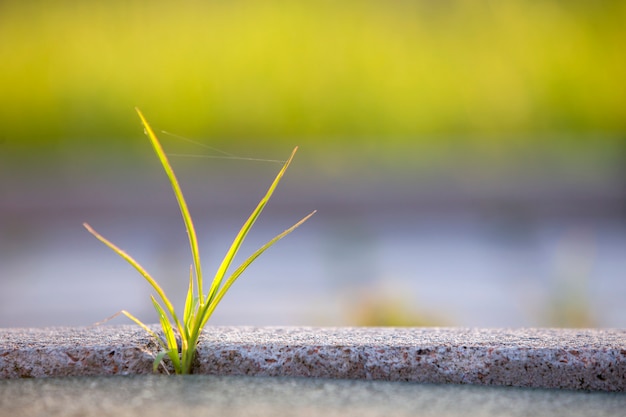A close-up portrait mode image captures a single grass sprout emerging from a tiny gap in a textured concrete pavement, speckled with white, gray, brown, and black. The sprout, consisting of eight distinct blades, stands vividly green with yellow highlights where the sun touches it. The lone plant is located on the left side of the image, bordered at the base by a blurred concrete curb that gives way to a hazy backdrop. Above the yellow-green upper third of the background, possibly indicating sunlit foliage, there lies a grayish, potentially a man-made structure such as a bridge, sidewalk, or road, though its exact nature is indistinct. A delicate spiderweb stretches between two of the grass blades, adding a subtle detail to this representation of resilience in an urban setting.